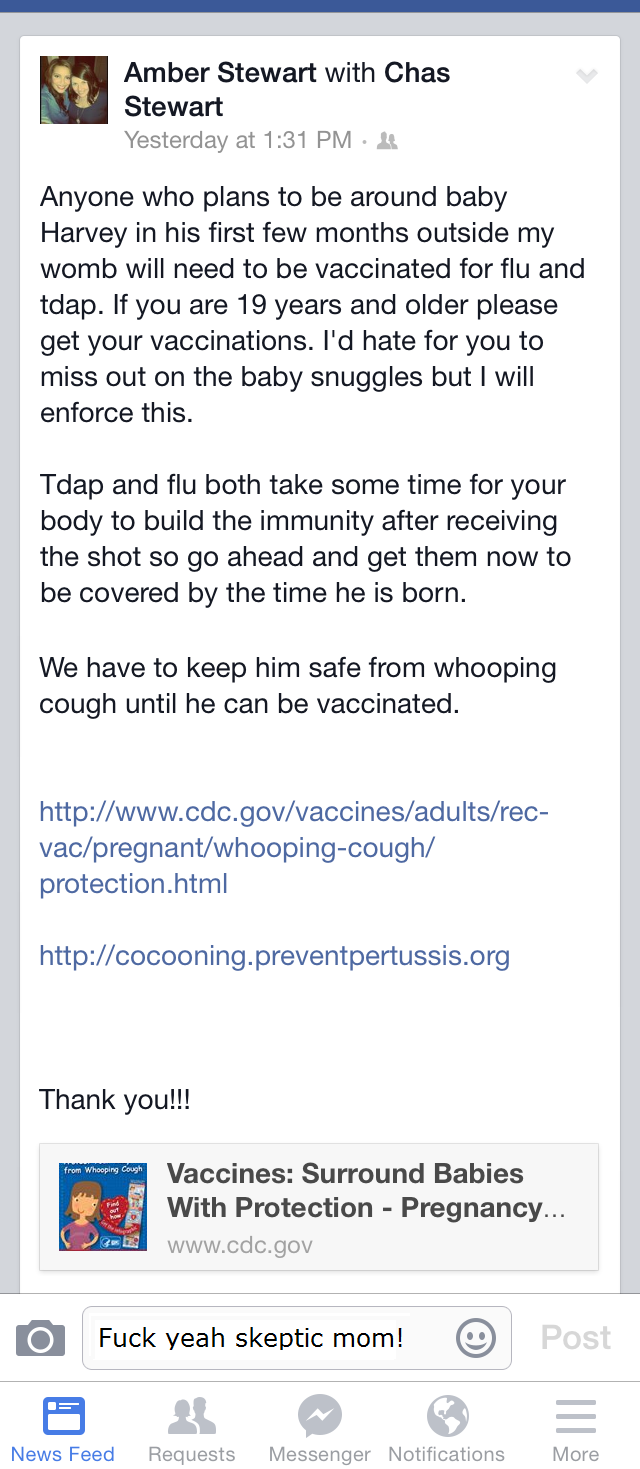Digital image shows two women, Amber Stewart and Chaz Stewart, in a cheerful profile photograph taken on [insert date based on "yesterday at 1:31 pm"]. Both women are smiling and appear happy. The image is accompanied by an important message from Amber Stewart, emphasizing the need for anyone planning to be around baby Harvey in his first few months to be vaccinated for flu and Tdap. She highlights the necessity of being immunized to protect the baby from whooping cough and mentions the cooldown period required for the vaccines to build immunity within the body. Amber provides links for further information from trustworthy sources, including the CDC (cdc.gov/vaccines) and cocooningpreventpertussis.org. She firmly states that while she values visitors' company, baby Harvey's safety comes first.